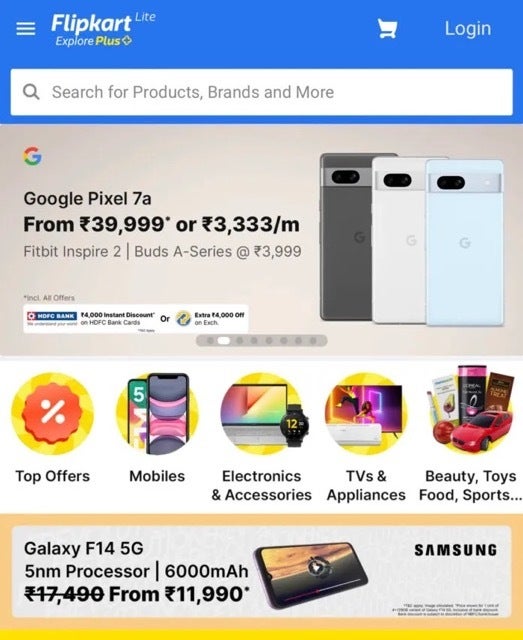This image is a cropped screenshot of the homepage of the Flipkart Lite website. The top of the screenshot displays a blue header. On the left-hand corner of the header, three white vertical lines are visible, signifying a menu icon. The website's logo, "Flipkart Lite Explore Plus," is prominent at the center. On the right-hand side, there are icons for a shopping cart and a login button, both in white. 

The header also contains a white search bar with placeholder text that reads, "Search your products, brands and more."

Below the header, the main body of the website is displayed, divided into three sections. 

The first section is an advertisement for the Google Pixel 7a phone, showcasing three images of the phone's rear view in different color options.

The second section features graphical images linking to various categories of the website, such as mobiles, electronic accessories, TVs, and appliances.

The third and final section is an advertisement for the Samsung Galaxy F14 5G phone.

Overall, the screenshot presents a concise view of the main elements on the Flipkart Lite homepage, focusing on product advertisements and site navigation options.